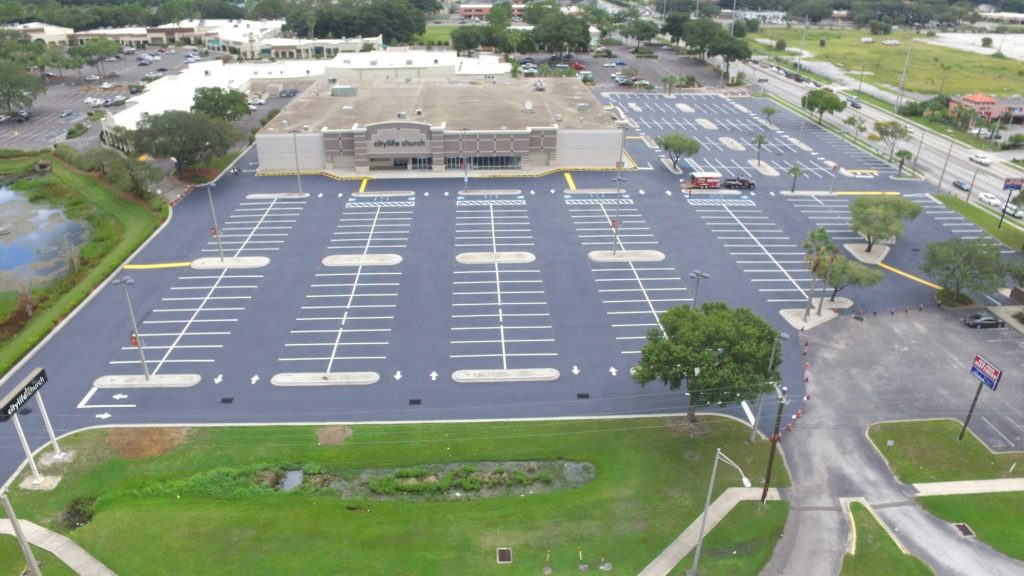The aerial photo captures a large, horizontally-aligned parking lot with distinct white lines marking the parking spaces. At the top of the image, just beyond the parking area, stands a single-level building with a beige and brown stone facade. This building has been converted into the City Life Church, as indicated by the signage on its gray-trimmed front. 

The church's structure includes a flat, dirty gray roof peppered with HVAC equipment. To the right of the building, the parking lot seamlessly extends, and within it, a lone truck with a trailer is parked. The lot itself is largely empty, save for some trees, and features curved roads at the bottom leading out of the area.

On the left side of the image sits a small pond with some brown debris floating on its surface. The background, particularly the upper left corner, shows additional single-level buildings and their accompanying parking lots with a few cars. Further back on the upper right, expansive grassy lands are visible, separated from the church's parking lot by a busy highway, featuring two lanes on each side. This detailed scene captures the juxtaposition of urban infrastructure against the quieter, green expanse beyond.